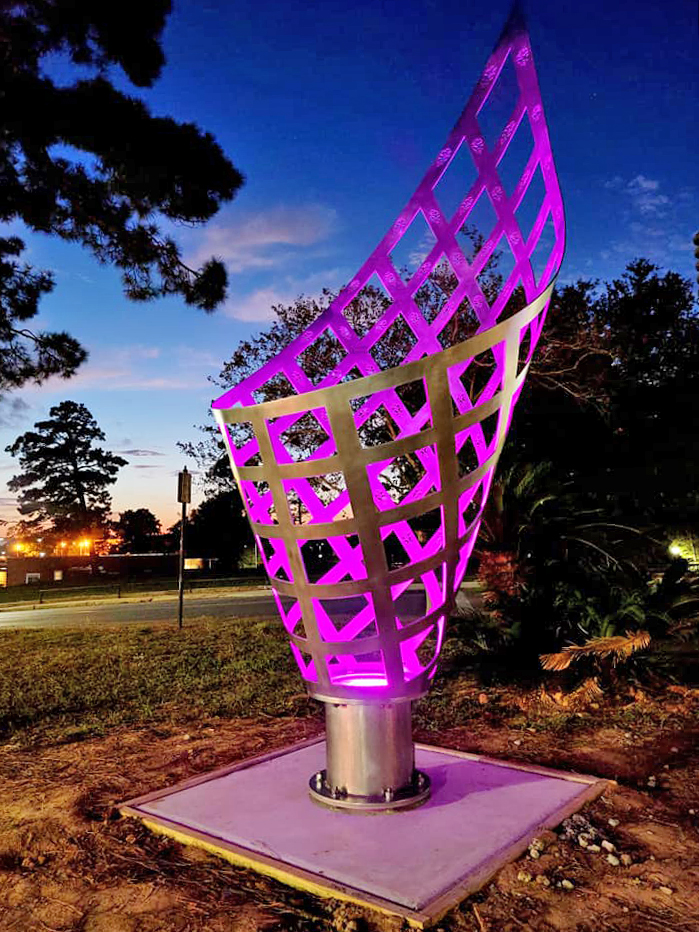The image captures a striking scene during twilight, with the sky transitioning from darker blue in the upper right corner to lighter hues towards the horizon, where sunlight beams through the trees. The centerpiece of the scene is a metal sculpture that evokes the shape of a flame or an ice cream cone, with a latticework design resembling a rolled chessboard or an upside-down lampshade. This structure is bolted to a cement base, and within its hollow, cone-like form, a powerful spotlight projects a vibrant lilac or bright pink light upwards, enhancing its ornamental presence. Surrounding the sculpture are patches of dirt, grass, gray rocks, and trees with green and brown leaves. Houses and lights are faintly visible in the background, completing the setting of this intriguing artwork illuminated against the dimming sky.